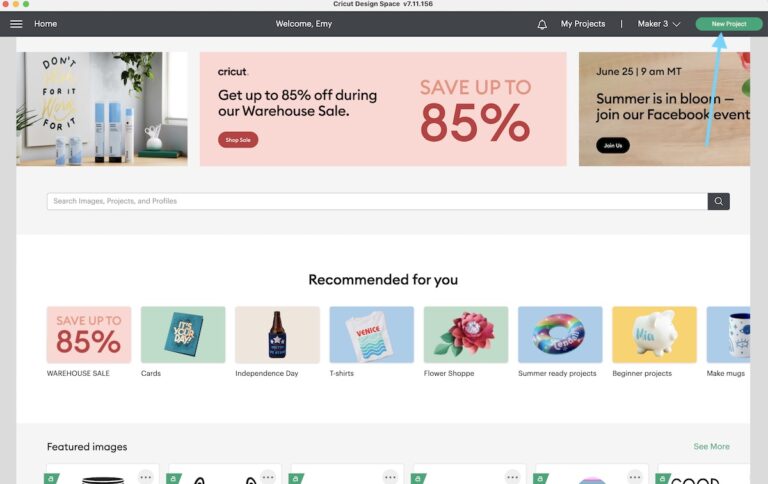The image appears to be a screenshot of a website displayed on an OSX operating system. In the top left corner, there are the typical OSX window buttons in red, yellow, and green for closing, minimizing, and maximizing the page, all set in a light gray bar. Below this is a dark gray navigation bar featuring a menu button on the far left, followed by the options: "Home," "Welcome, Emmy," a notification bell, "My Projects," "Maker 3," and a prominent green button with white text that says "New Project," accompanied by a blue arrow pointing to it.

The main content area of the webpage is divided into several sections. At the top, there appear to be banner ads, including an image potentially showcasing skincare products. There's a noticeable red box announcing a "Cricket" warehouse sale with up to 85% off, labeled "Shop Sale" in red text. Additionally, another promotion on the right mentions an event: "June 25th, 9 am MT, Summer's in Bloom, join our Facebook event," though the text is cut off.

Below this section, there is a search bar labeled "Search images, projects, and profiles." Underneath the search bar is a section called "Recommended for you," which includes various thumbnails with labels such as "Save up to 85% Warehouse Sale," "Cards," "Independence Day," "T-Shirts," "Flower Shop," "Summer Ready Projects," "Beginner Projects," and "Make Mugs." This section appears to continue but is cut off in the image.

Further down, there's a section titled "Featured Images," though the details are also cut off. However, there is a visible green link on the right side that says "See More."